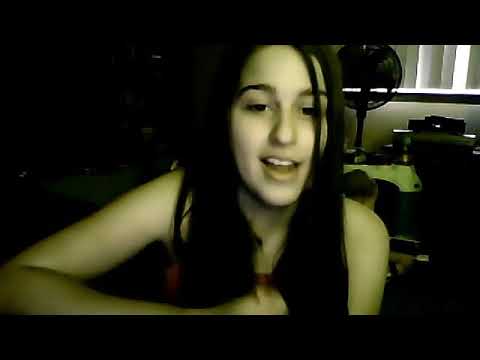The photograph captures a young woman with long, dark hair and olive skin, looking directly into the camera and smiling, with her mouth slightly open as if she's in the middle of speaking. She is wearing a sleeveless blouse and has one arm lifted with her hand in front of her chest, while her other arm rests by her side. Her hair falls past her shoulders, with one strand partially covering her eye. The image has an olive-green tint and is framed with black bars at the top and bottom, resembling a cinematic format. The setting is a dimly lit room, appearing almost underexposed, particularly on the left where details are obscured by darkness. On the right side of the image, there's a partially illuminated window with closed Venetian blinds, through which a little light filters in. Below the window, a black metal fan sits on what seems to be a desk cluttered with indistinct objects. A chair is also faintly visible in the background.